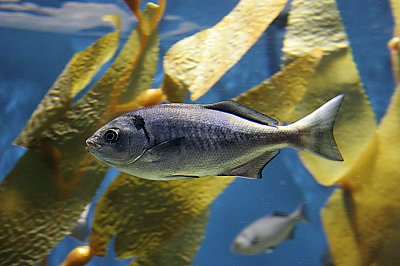This image is a detailed, close-up photograph of an aquatic scene centered on a small, grayish-blue fish. The fish, with its distinct eye and slightly open mouth, swims prominently in the middle of the frame, moving towards the left. Its scales form a gradient of gray, and its small fins and typical tail are captured clearly. Surrounding the fish are strands of yellowy-golden green seaweed, waving through the blue water. Behind this primary fish, blurred in the background, is another fish of the same species, adding depth to the scene. Additionally, a smaller orange fish appears in the bottom left-hand corner, providing a contrast to the dominant gray hues. The vibrant blue water serves as a serene canvas, amplifying the colors and details of both the fish and the seaweed in this underwater snapshot.